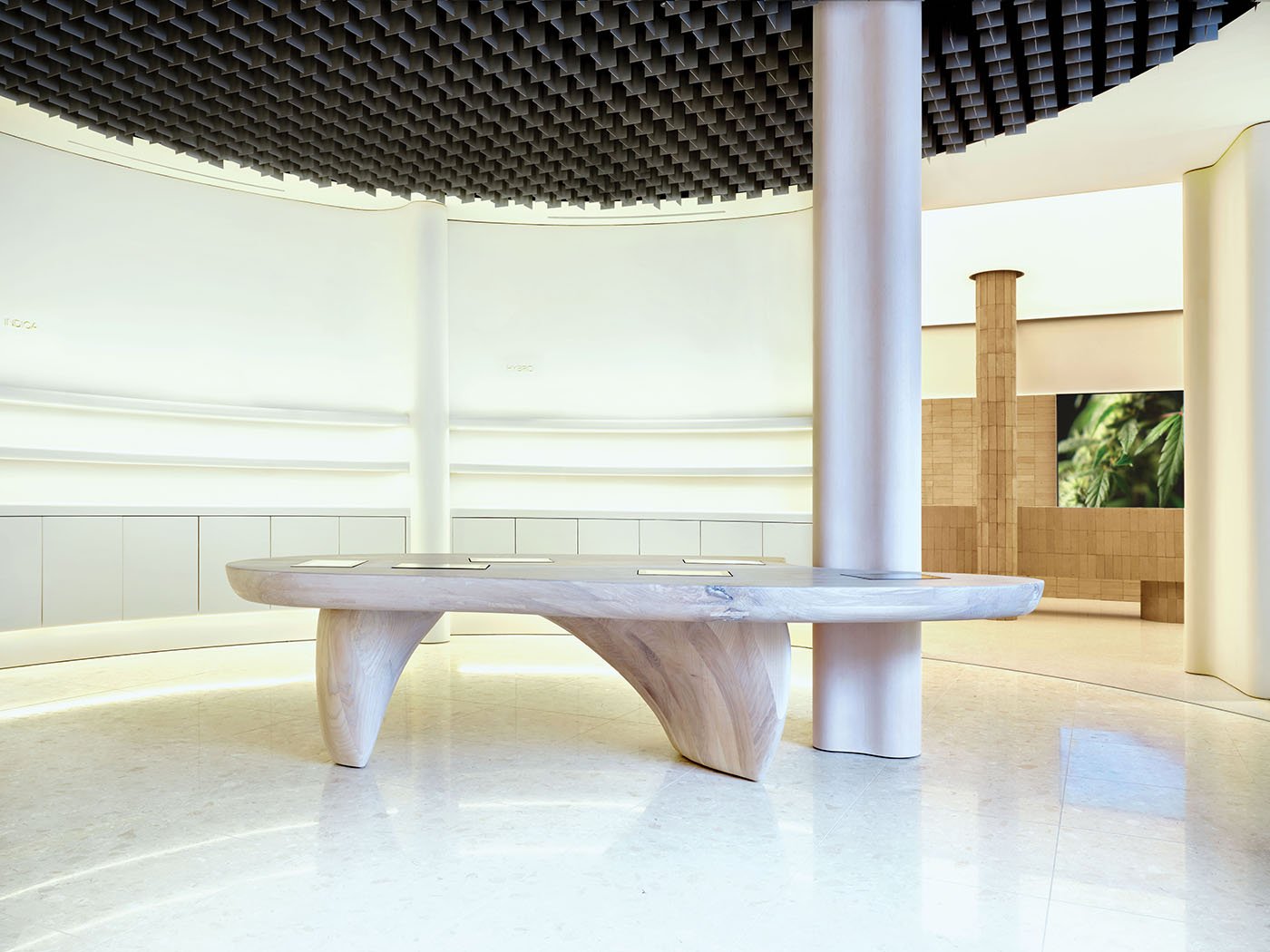The image depicts a modern, enclosed outdoor patio characterized by its striking architectural features and sleek design. The focal point is a uniquely designed wooden table, with one leg significantly wider than the other, and several pieces of paper, possibly menus, resting on its surface. To the right of the table stands a white pillar extending up to the ceiling, which has a honeycomb-like texture with small holes. The shiny, white floor mirrors the room's minimalist aesthetic. The background reveals a glass enclosure, with visibility partially obstructed by foggy windows, a TV screen or artwork, and another pillar. The walls are pristine white, and on the right side of the image, there appears to be a staircase leading downwards, potentially to a gift shop. The ceiling features a cool black texture, contrasting with the overall light color scheme. The adjacent room, visible in the background, has tan walls, a large window, and lush green leaves peeking through.